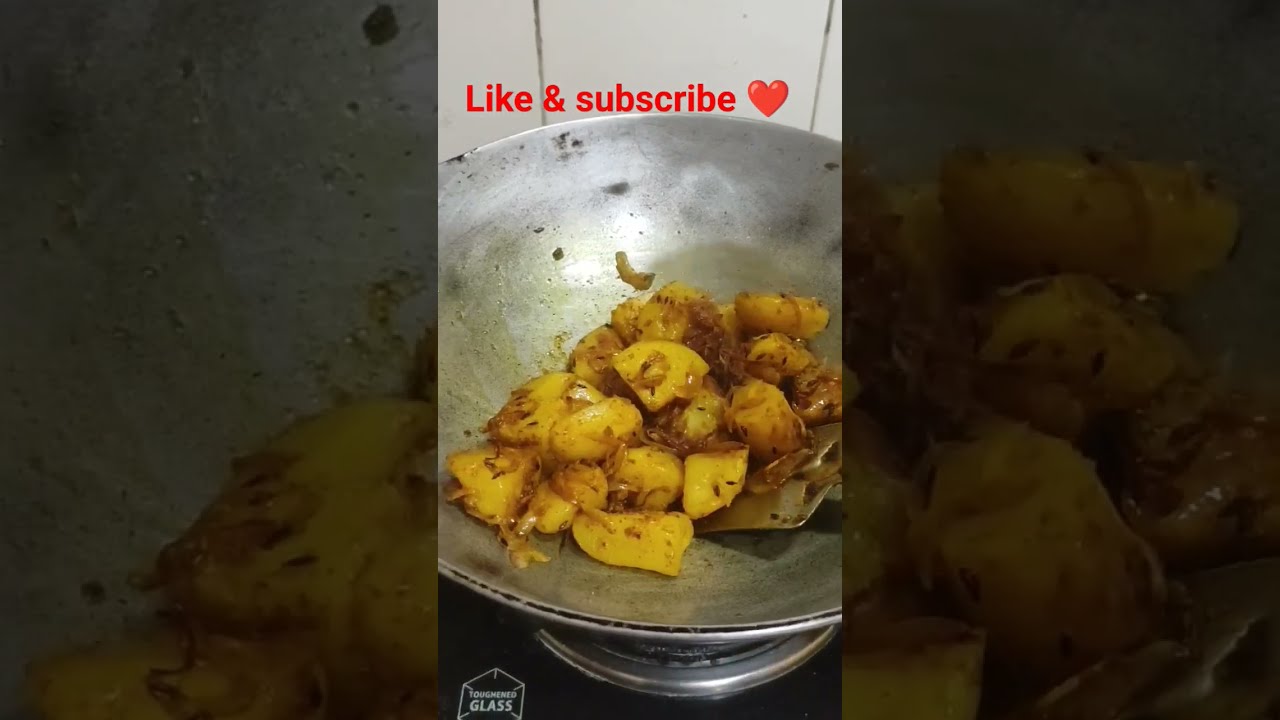This image consists of a horizontal rectangular layout with three adjacent vertical panels. The central panel, a narrow vertical rectangle, is the primary focus, featuring the prominent text "Like and Subscribe" at the top in red, accompanied by a red heart icon. Below this text, there is a large, metallic wok filled with chunks of yellowish, brown-topped food that appear to be potatoes, although they could also be plantains with a brown glaze or spices sprinkled over them, hard to discern exactly. The wok sits atop a black surface, possibly a stove or counter, conveying a cooking setting. At the bottom of the central panel, a small white icon in the shape of a hexagon displays the text "toughened glass". Flanking the middle panel are two wider vertical rectangles, each featuring a zoomed-in, darker, and more faded close-up of the food and parts of the wok, serving as a subtle background extension of the central image. This composition, rich in shades of red, brown, and metallic silver, suggests an active cooking scene, possibly within a home kitchen, and hints at a social media context where the call-to-action "Like and Subscribe" implies the image might be from a cooking video or livestream on platforms like Instagram or TikTok.